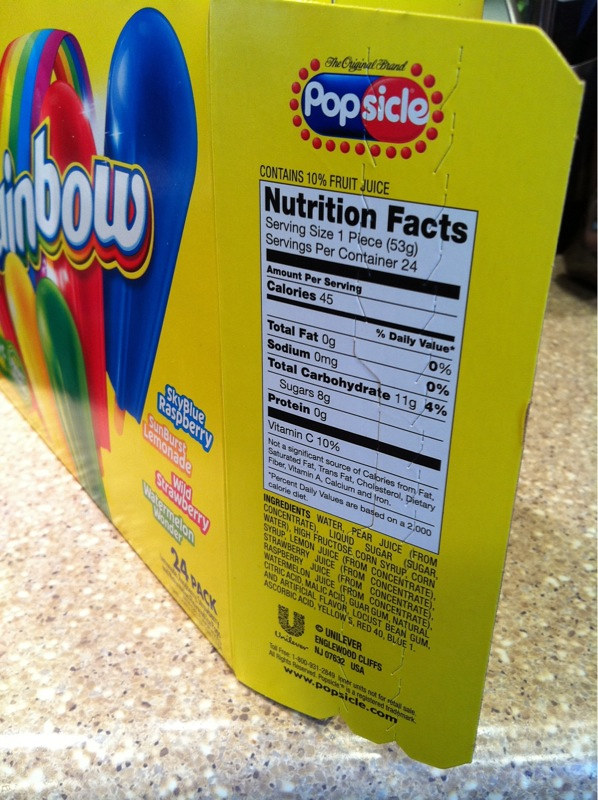A brightly colored box of Rainbow Popsicles rests on a light gray granite countertop. The box is primarily yellow with vibrant images of the popsicles, which come in sky blue raspberry, strawberry lemonade, wild strawberry, and watermelon flavors, depicted in blue, yellow, red, and green hues respectively. Prominently displayed on the side of the box are the nutrition facts, which are printed in black letters on a white background.

Each popsicle serving is 53 grams, with the box containing a total of 24 servings. The nutrition label reveals that each popsicle contains 45 calories, 11 grams of total carbohydrates (4% of the daily value), including 8 grams of sugar, and offers 10% of the daily recommended intake of vitamin C. The ingredient list starts with water and pear juice among other components, and it notes that the product is manufactured by Unilever, the same company known for making deodorants. This detailed image emphasizes the nutritional information and branding of the Rainbow Popsicles.